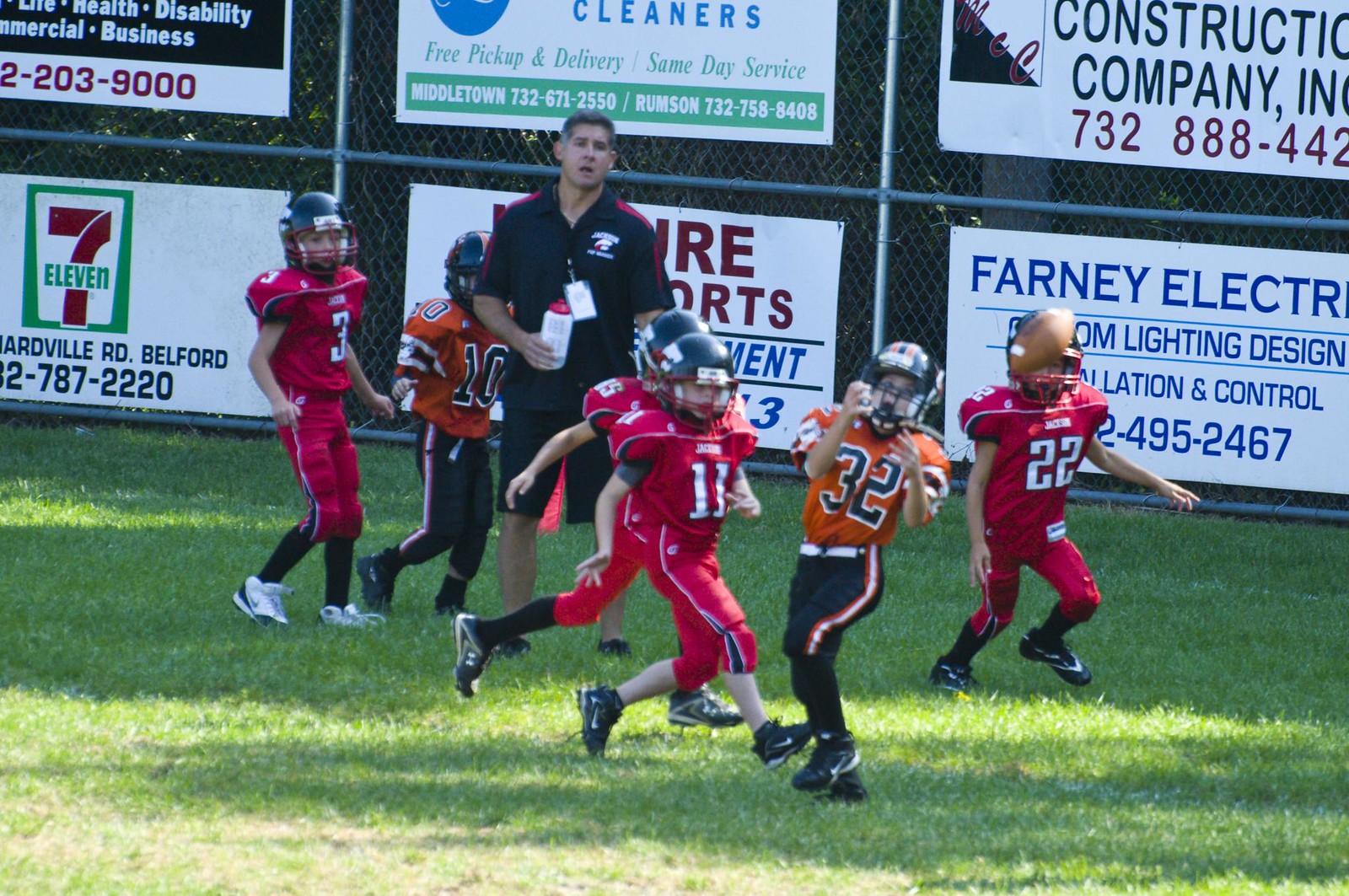In the image, six children are engaged in a lively youth American football game on a lush green field. The players are divided into two teams; four of the children are dressed in red jerseys with black pants, sporting numbers 3, 11, 22, and a partially visible number ending in 5. The remaining two children wear orange jerseys—number 32 with black pants and number 10. The player in the red jersey marked with 22 is captured with a football directly in front of his helmet. To his left, player number 32 in an orange jersey is poised to catch the ball. A man, presumably a coach or referee, stands attentively behind the players. He’s dressed in a dark blue shirt and blue shorts, holding a white cup with a red lid, and wears a lanyard with a white card around his neck. His grayish hair and slightly open mouth suggest he’s calling out or giving instructions. Behind him, a metal-wire fence features several advertisements, including those for Farney Electric, a construction company, a cleaners offering free pickup and delivery, and a 7-Eleven. The sun highlights parts of the grass, casting shadows and adding to the vibrancy of the scene. The atmosphere is energetic and the day appears to be beautifully bright.